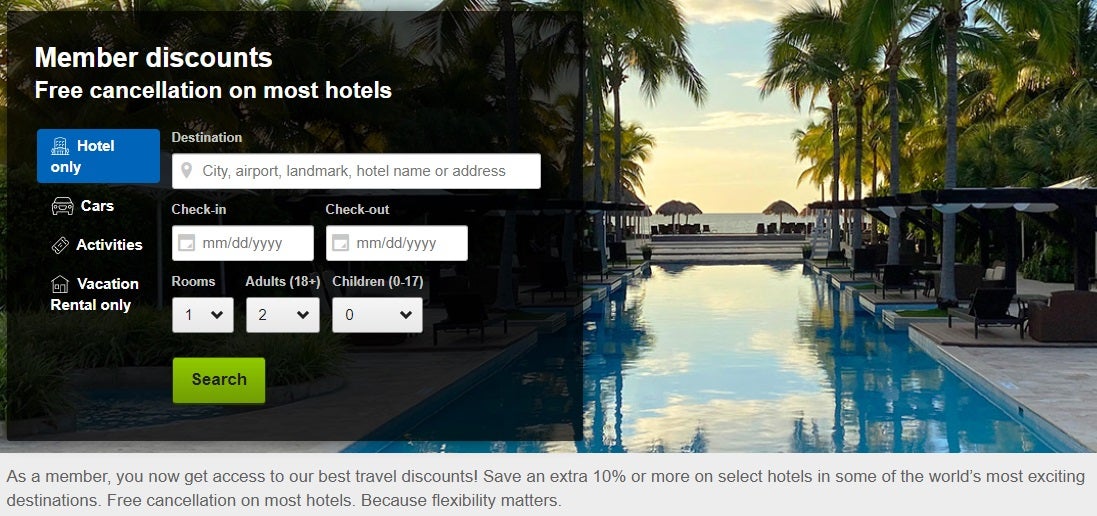An image displays a sleek and sophisticated travel website interface, featuring a vibrant picture of a luxurious resort pool framed by lush palm trees with the ocean glimmering in the background. Key elements include a search bar for inputting your destination, check-in and check-out dates, the number of rooms, adults, and children. There are options for reserving cars and exploring various regional activities. Additionally, users can find vacation rentals if they prefer not to stay in a hotel. Prominently, the website advertises special member discounts, highlighting benefits like free cancellations on most hotels, due to the importance of flexibility. At the bottom, it states that members will now gain access to the best travel discounts, with an extra 10% savings or more on select hotels in some of the world's most exciting destinations.